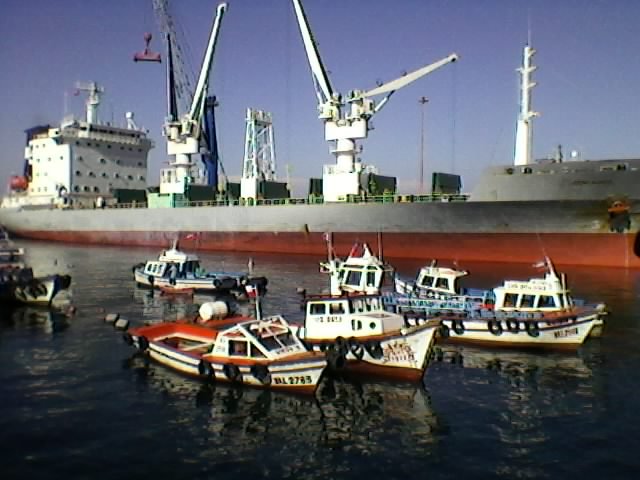A bustling scene unfolds on the dark, choppy waters of what appears to be the ocean. Dominating the entire background is a massive cargo ship, possibly a Navy vessel or an aircraft carrier, with a striking gray body and a burgundy line along its waterline. The vessel, adorned with various towers and cranes, stretches across the full length of the image under a solid blue sky.

In stark contrast to the colossal ship, a group of around six to eight much smaller boats congregates closely in the foreground. These boats, which could be tugboats, fishing trolleys, or even police boats, are primarily white with accents of red and blue. Each small boat is detailed with three windows and life rings attached to their sides, and they are equipped with small black circles that might be portholes or fenders. Most of these boats seem to be drifting towards the left, while one ventures to the right. The compact formation of the boats and their significant size difference compared to the cargo ship create a dynamic and intriguing maritime scenario.